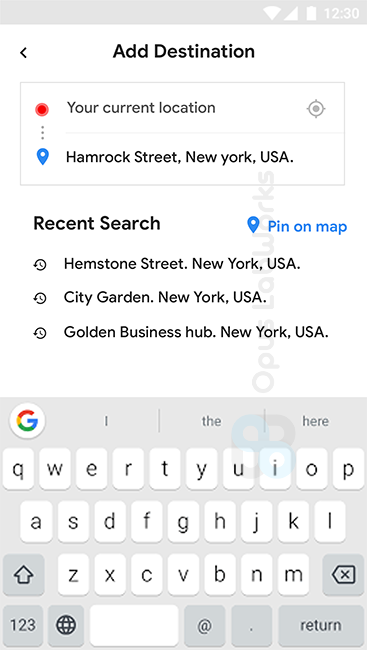The image displays a smartphone screen showcasing a navigation app. At the top, there's an option to "Add Destination," followed by a section displaying "Your Current Location" and the address "Hamrock Street, New York, USA." Below this, under "Recent Searches," there is a clickable link labeled "Pin on Map" highlighted in blue. Further down, the recent search history includes "Hemstone Street, New York, USA," "City Garden, New York, USA," and "Golden Business Hub, New York, USA."

At the bottom of the screen, Google’s colorful 'G' logo appears next to a text input field that begins with "I the here." The background of this lower section is a gray rectangle, containing a virtual keyboard. The keyboard features alphanumeric keys, a globe icon for language selection, a backspace key, a return key, an '@' symbol, and a period/full stop button along with a space bar. The overall layout is typical of a modern smartphone navigation interface, providing easy access to recent destinations, search functionalities, and input options.